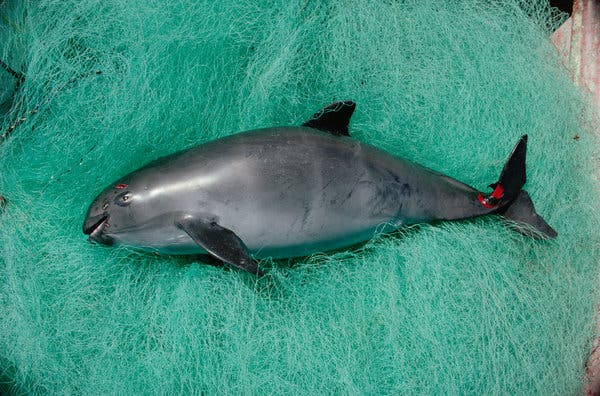The image features a horizontally aligned, large, and mostly silver-gray fish with blue tints on its side. The fish is centered perfectly within the composition, lying on a backdrop of light green netting that fills most of the background. The fish's mouth is slightly open and faces left, while its narrower tail points to the right. The tail fin is small, with one side gray and the other black. The fins located on its sides are darker, with a mix of silver and black on top. The fish has a wide body that gradually narrows towards its tail end, and its eye is open. There are also distinct details such as a red mark where the body connects to the tail and some ink-like markings on the bottom left side of the fish. The intricate netting beneath the fish is described as having a dense, almost foam-like texture with numerous fibers, contributing to the overall texture and depth of the image. Additionally, in the upper right and lower left corners of the frame, there are visible hints of other colors and shapes, including pink, gray, and black.